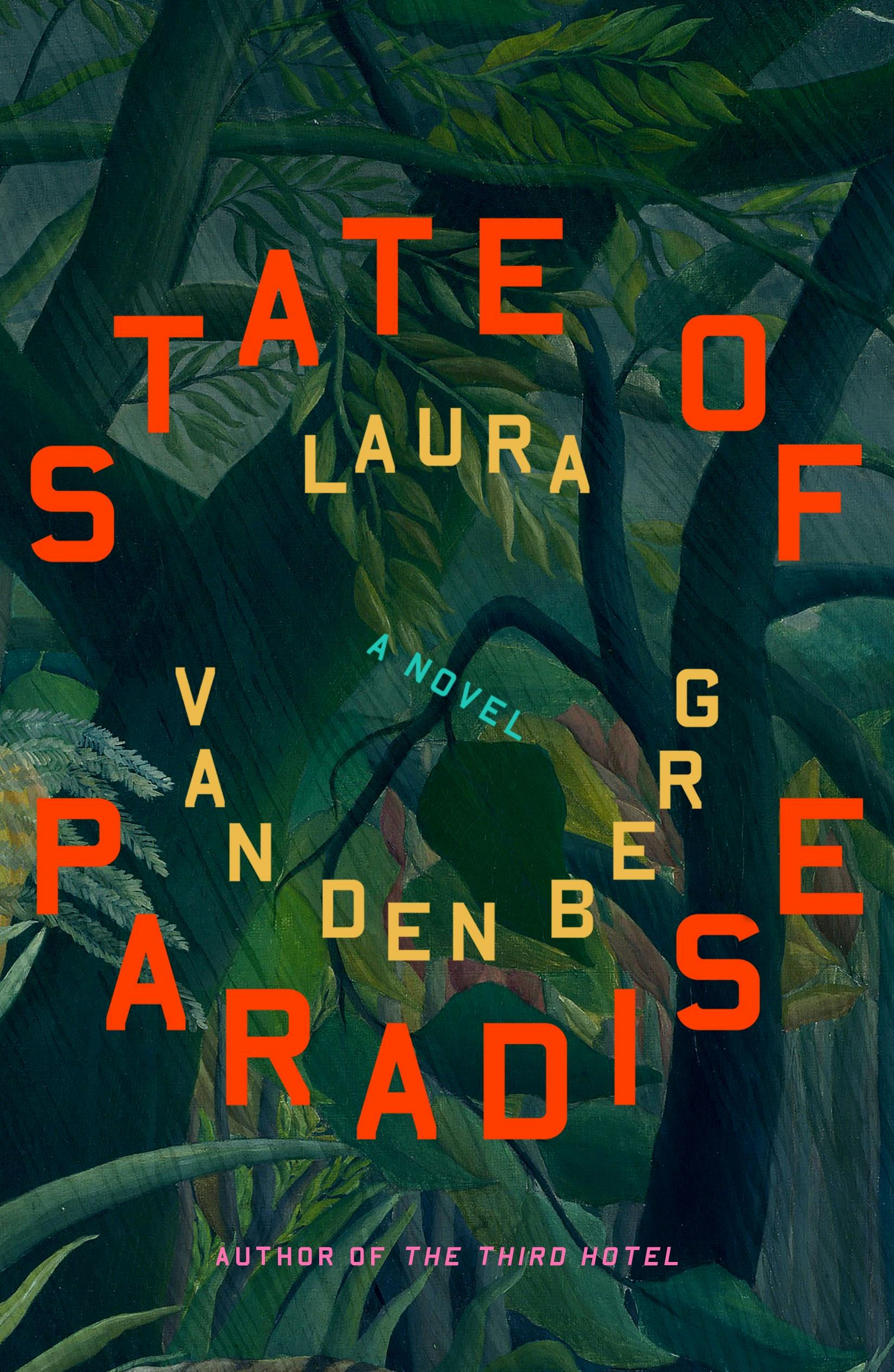The image showcases the cover of Laura Vandenberg's novel "State of Paradise." The title "State of Paradise" is prominently featured in large, bold red letters arranged in a circular pattern. Encircling the title, the author's name, Laura Vandenberg, is written in a yellowish-gold font. Inside this circle, in smaller bluish-green letters, the phrase "a novel" can be found. At the bottom of the cover, in pastel pink letters, it states "author of The Third Hotel." The background is an artistic rendering of a forest, with various shades of green leaves and brown tree trunks, suggesting a rainy scene with rain appearing to fall sideways to the right.